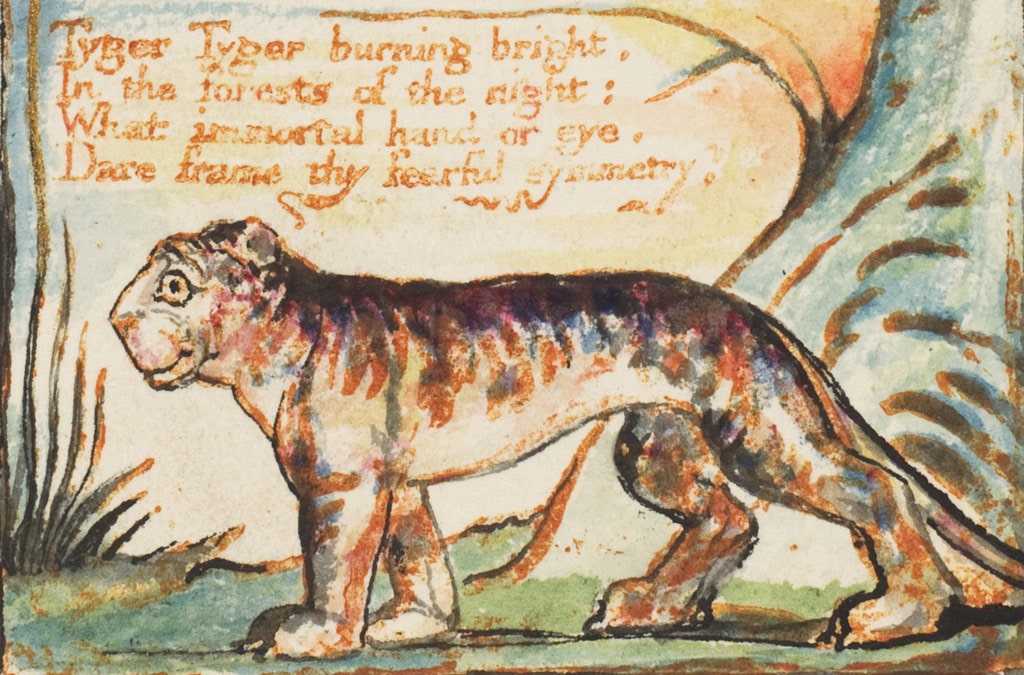This vibrant painting, possibly an illustration from a children's book, vividly portrays a tiger standing on all fours and facing left. The tiger, depicted with a somewhat cute and smiley expression, is set against an abstract background featuring a tree trunk on the right and some grass on the left, with hints of a field or a hill. The artwork is accompanied by handwritten text at the top, quoting the famous verse: "Tiger, Tiger, burning bright, in the forests of the night, what immortal hand or eye, dare frame thy fearful symmetry?" Although possibly misattributed to Rudyard Kipling, the lines are from William Blake's poem "The Tyger."